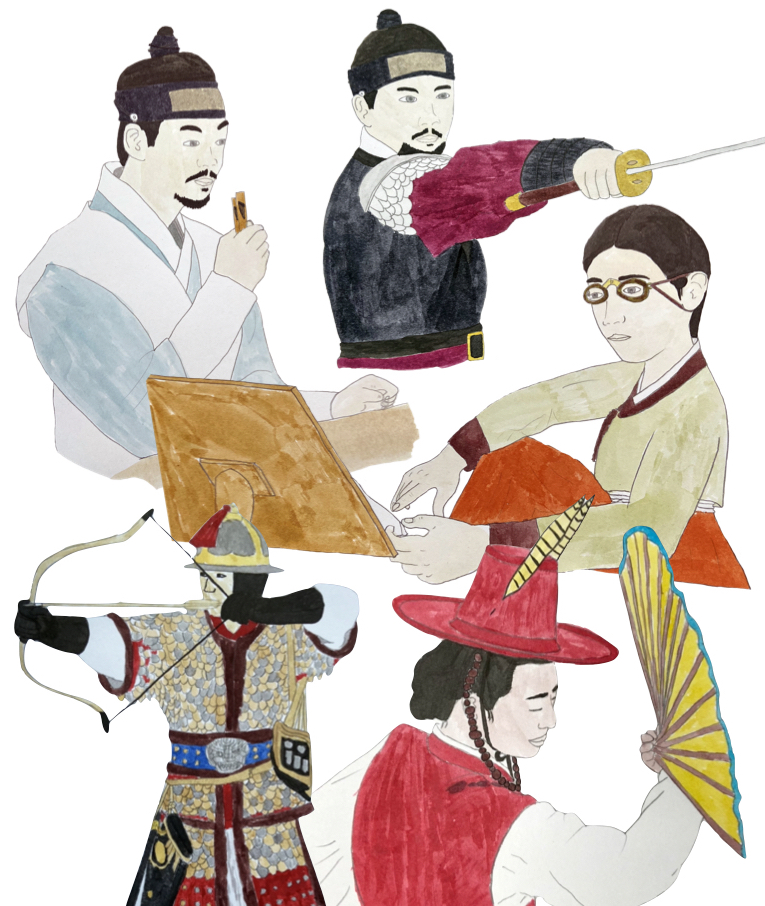The image is a detailed, colored pencil drawing portraying a variety of Asian figures with distinct roles and traditional attire. On the right, a bearded warrior in a blue and white outfit with a cap holds up an item as if about to eat it. Next to him, another warrior brandishes a sword, wearing a black vest with a gold buckle, a red elbow-length glove, and a matching cap. Below, a man with glasses and short hair, dressed in a gray shirt and red pants, appears engrossed in reading. On the left, a traditional archer pulls back his bow, adorned in ancient garb with black gloves. Finally, to the right, a dancer in a red hat with feathers, a red vest, and a white shirt gracefully holds a yellow fan edged with teal. The overall aesthetic features watercolor-like outfits in shades of light blue, black, gold, silver, and red, emphasizing their diverse roles and cultural attire.